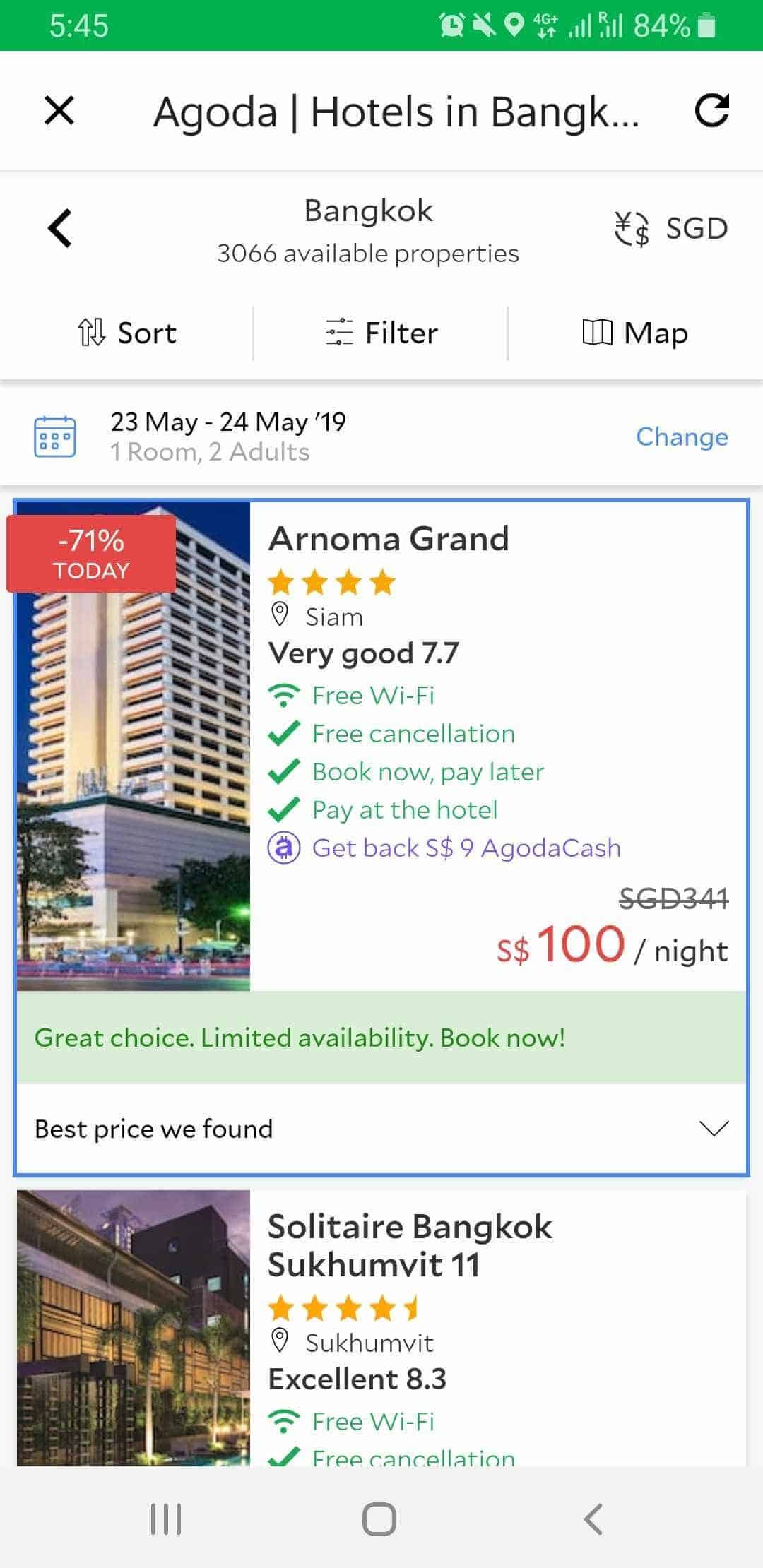In the screenshot of a mobile device, the time displayed in the upper left corner is 5:45. The upper right corner features several status icons, including an alarm icon, a news icon, a location icon, a 4G network indicator with full signal strength (4 out of 4 bars), and a battery icon showing the battery level at a critical 4%. The screen displays the Agoda app, highlighting hotel options in Bangkok. The search results show 3,066 available properties. Two highlighted listings include the Anomal Grand, rated 4 stars with a "Very Good" rating of 7.7, and the Solid Tie Bangkok, rated 4.5 stars with an "Excellent" rating of 8.3. Additional perks listed for these hotels include free Wi-Fi and free cancellation options.